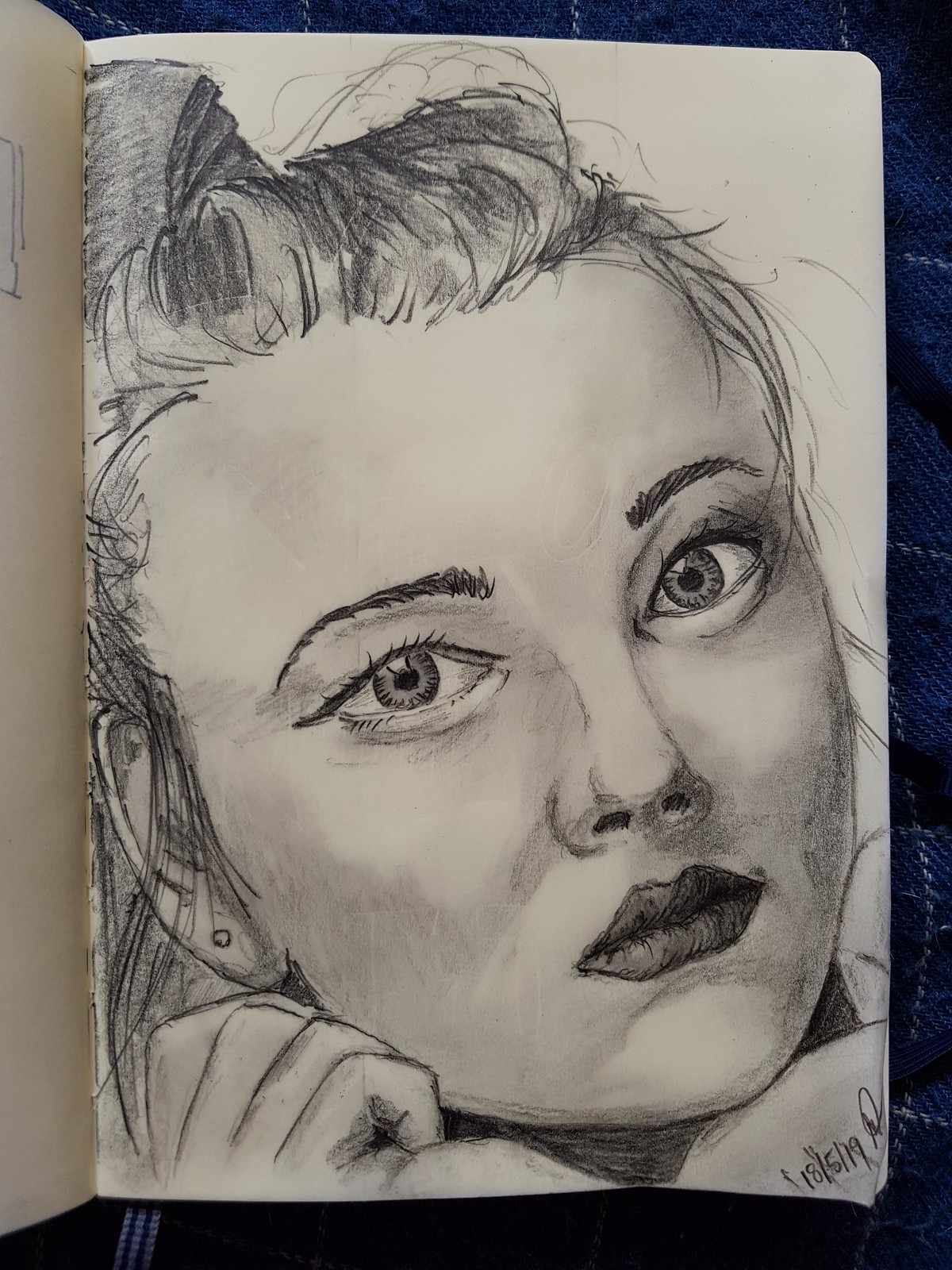A detailed graphite pencil sketch portrays the face of a woman with distinctly feminine features. Her hair, meticulously shaded in black and white, suggests voluminous curls with bangs gracefully cascading over her left eye. The shading technique enhances the texture, highlighting the intricate curls and reflective quality of her hairstyle. Her eyes, large and expressive, are the focal point, rendered with careful shading to indicate reflections, although the absence of color leaves their hue to the imagination. 

Her facial features are well-proportioned, with full lips and closed mouth, framed by dark, meticulously shaded eyebrows that add to her expressive look. A small circle stud, representing an earring, adorns her ear, subtly enhancing the portrait's detail.

The artwork appears on a page from an artist's sketchbook, characterized by a seamless edge rather than a perforated, ring-bound one. The sketchbook lies on a piece of fabric featuring a predominantly blue hue, accented with black and white checkerboard pattern details. At the bottom of the page, there is a date inscribed as "18/5/19" accompanied by initials that are not clearly legible, indicating when the sketch was completed.